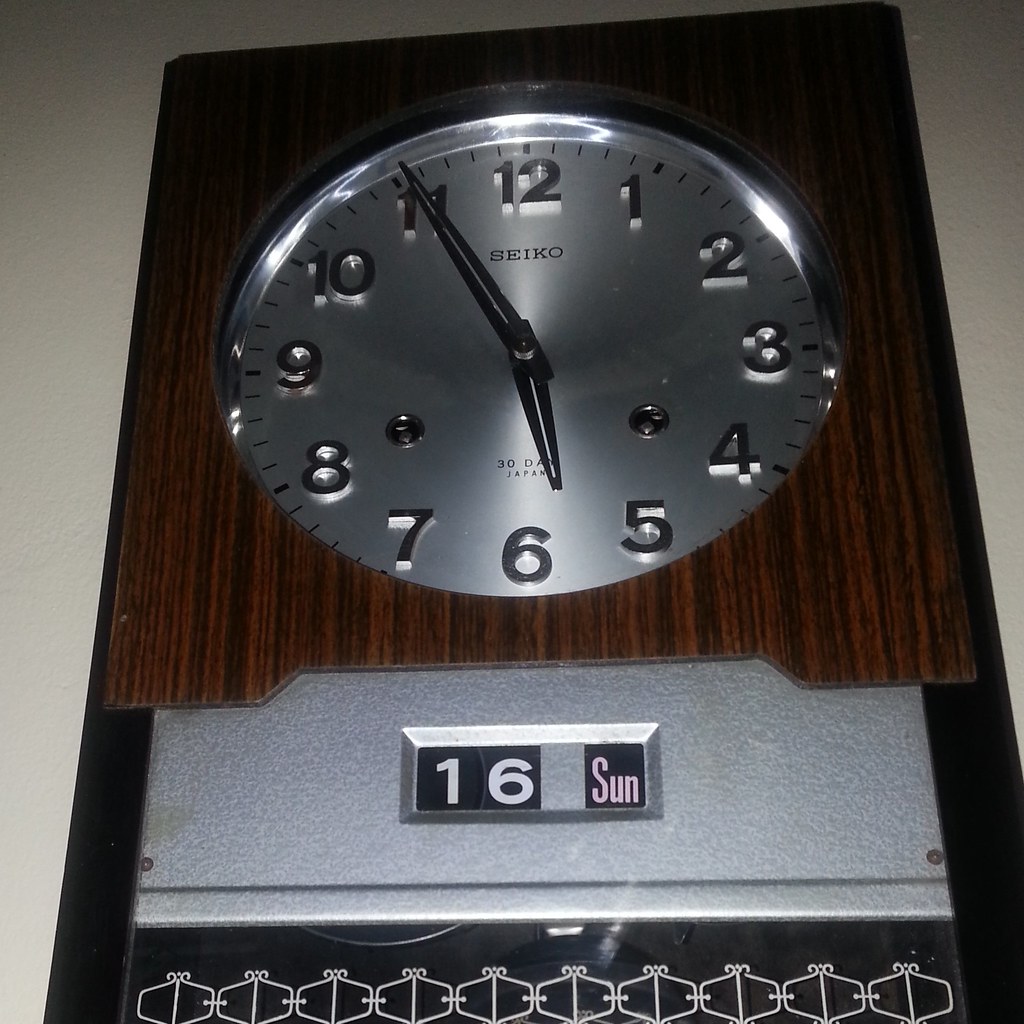This close-up photograph captures a vintage Seiko 30-day analog wall clock set against a beige or whitish-gray wall. The clock is rectangular in shape and features a visually striking design with various materials and colors. The lower portion of the clock includes a dark wooden section with vertical grain and a black border adorned with white oval-like symbols. Above this is a speckled, metallic silver surface that hosts a raised area labeled "16 SUN," indicative of a date mechanism with numbers that likely flip over.

Moving upwards, the clock transitions into a section of dark green wood, also with vertical grain, framing a circular clock face. The clock face itself is silver, marked with black numerals from 1 to 12 and black minute dashes. The hands of the clock, indicating approximately four minutes to six, are also black. The branding "Seiko 30 Day" and "Japan" appears below the hands. The clock also features two keyholes, one above the 4 o'clock position and one above the 8 o'clock position, for winding the mechanism. This detailed, multi-material timepiece combines both elegant and functional elements, making it a distinctive wall clock.